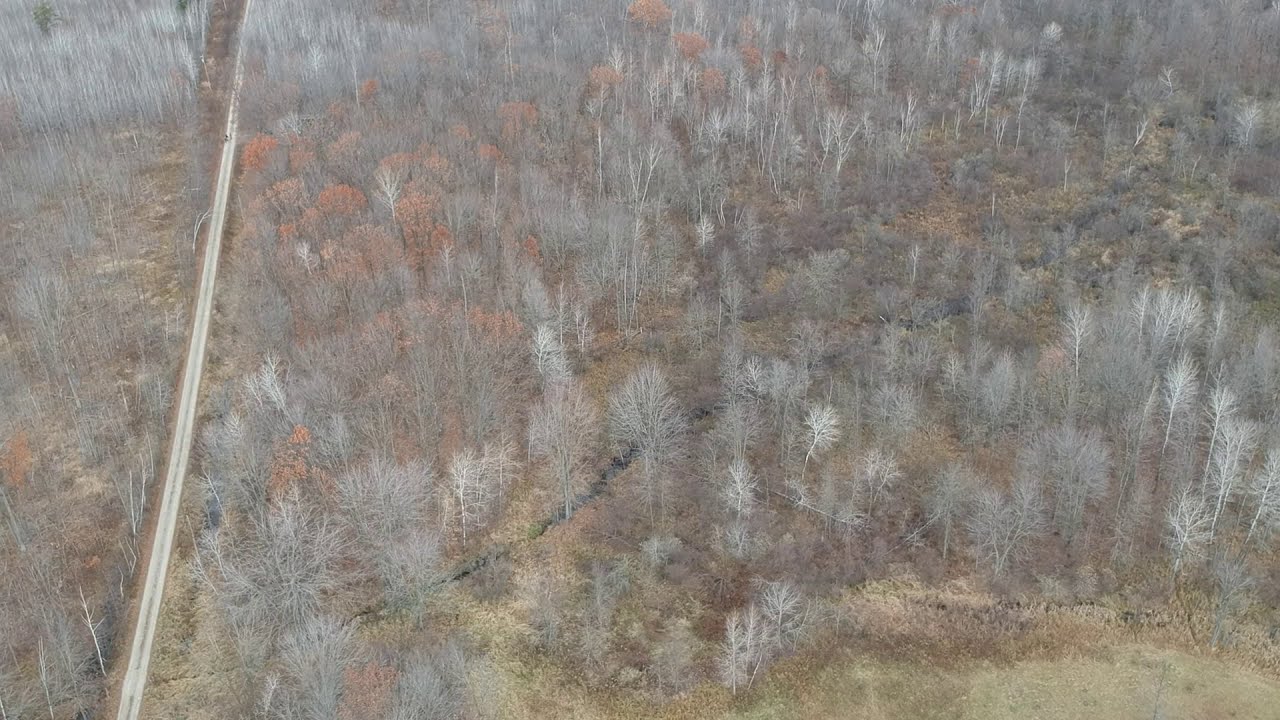The image depicts an aerial view of a forest, resembling a painting with its muted tones and stark details. Dominating the landscape are densely packed, leafless trees, casting a desolate and wintery atmosphere over the scene. A narrow, gray two-lane road cuts through the forest on the far left side, while a small stream weaves from the upper right-hand corner to the lower left-hand corner.

The trees, mostly gray and bare, give off a feeling of barrenness. Some trees retain a few leaves in shades of light green and orange, suggesting the transition between fall and winter. The ground below is a mix of yellow, brown, and tan hues. Pine trees are scattered throughout, adding slight variation to the otherwise monochromatic color palette. The overall effect is a rural, isolated wilderness, with the lonely road and subtle waterway adding to the sense of quiet desolation.